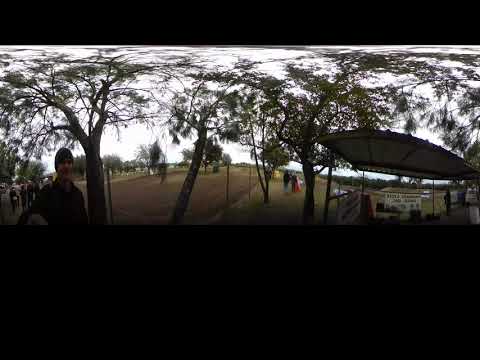In this highly distorted daytime photograph, the image appears to have been heavily manipulated, giving it a warped, stretched effect, reminiscent of a flattened 360-degree view. The scene is dominated by a white sky, beneath which tall trees with green leaves are bent and twisted, accentuating the photo's unnatural distortion. 

In the foreground to the left, a light-skinned gentleman wearing a dark top and possibly a hat looks directly at the viewer while holding a pole, likely a camera accessory. He stands near an open area resembling a market, populated by people walking around. The individuals are dressed primarily in darker clothing, though a few wear lighter attire. All appear somewhat blurred, indicating motion or further effects of the image manipulation.

Across the middle ground, there's a noticeable walkway where more people are mingling. To the right, a corrugated steel awning covers a market stand, beneath which an unreadable sign is positioned, accompanied by another sign to its left. The ground transitions from a brown field on the left side of the photo to more open grass areas.

Framing the image are two horizontal black bars, one thin at the top and a significantly larger one at the bottom, adding to the squeezed and compressed appearance of the photograph. The overall atmosphere suggests an overcast and colder day, with colors predominantly featuring tans, browns, dark greens, grays, some white, and hints of red.